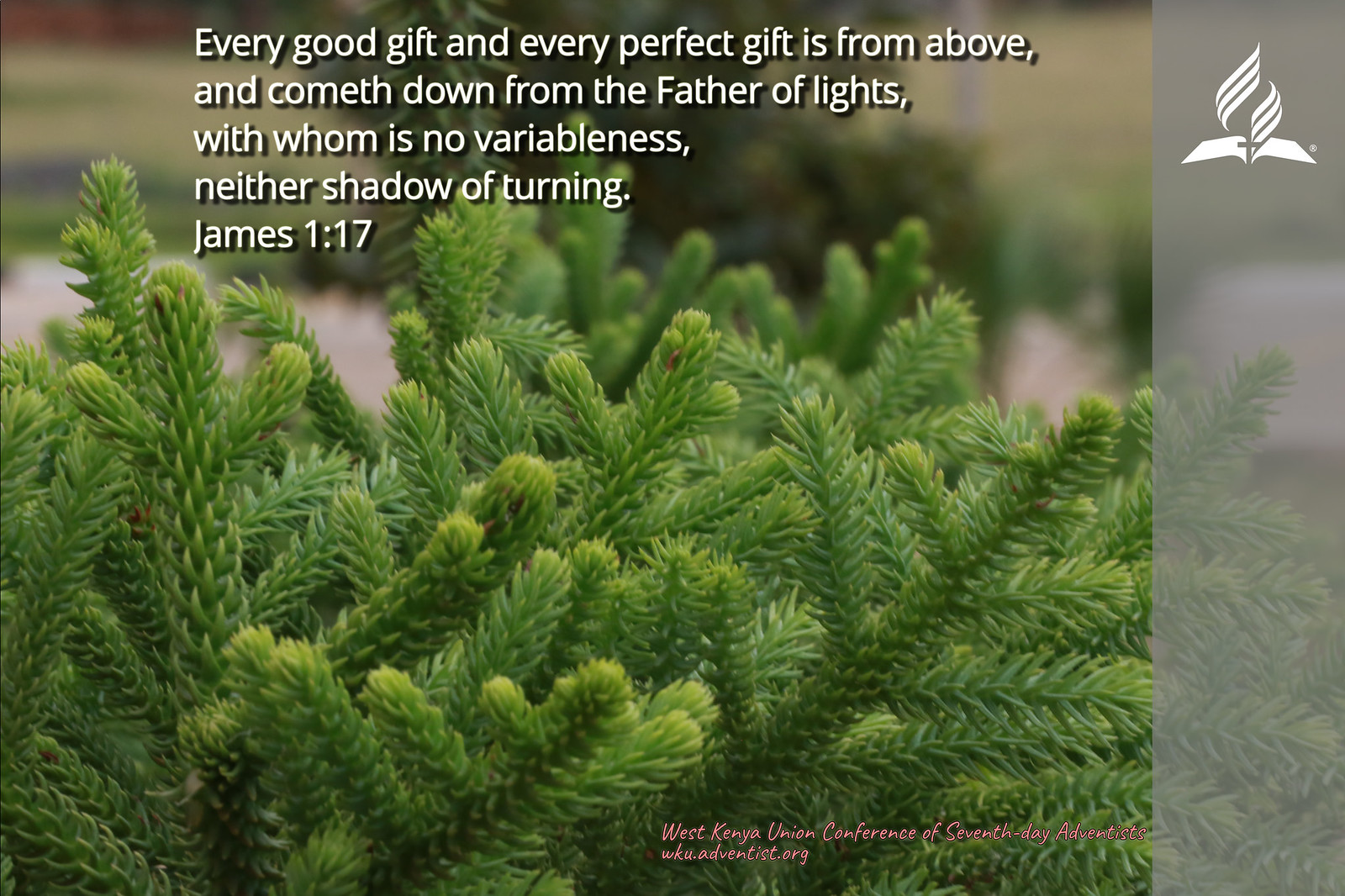This detailed photograph captures an unusual plant, closely resembling a bush with short, pine-like needles, or perhaps a cactus more than an evergreen tree. Superimposed on the image's varied texture of green foliage is Christian text in white, located in the top left corner. It reads: "Every good gift and every perfect gift is from above, and cometh down from the Father of lights, with whom is no variableness, neither shadow of turning, James 1:17." Adjacent to this text, in the top right corner, is a white logo depicting a Bible, a cross, and a symbolic flame. The bottom right section of the image features small pink text which states: "West Kenya Union Conference of Seventh-Day Adventists, wku.adventists.org." Additionally, the right side of the photo is partially overlaid by a gray bar.